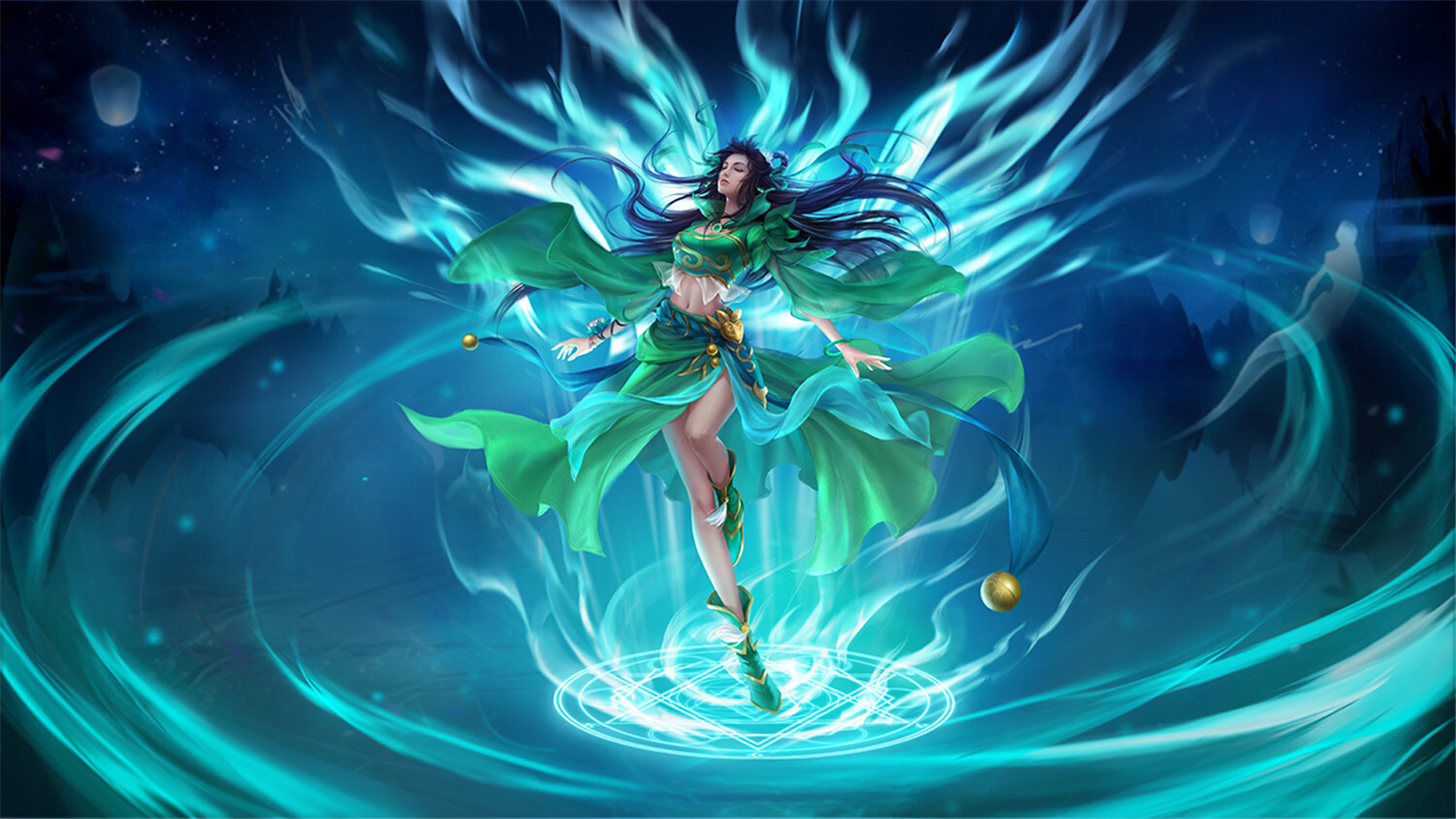The image is a highly detailed and expertly rendered piece of artwork, potentially from a graphic novel or video game, depicting an ethereal goddess-like character soaring through the night sky. The background features a whirlwind of blue hues with starry accents, evoking a sense of celestial wonder. Emerging from the center, the woman is adorned in an elaborate outfit consisting of a flared green and blue skirt and a crop top, which tastefully exposes her waist. Her striking, long, black-purple hair fans out behind her, with her eyes serenely closed and her arms at her sides.

Her ensemble is completed with green and gold boots that extend just above her ankles, and she wears a gold and blue belt with an emblem at its center. Above and below her, light blue and white auras contribute to the mystical atmosphere, with rays extending from her body like a radiant sun. Additional green, light green, and gold spiral swirls encircle her, further enhancing the dynamic and flowing nature of the piece. Distinct elements such as a gold sphere at the end of her gown and white streaks swirling beneath her boots add to the sense of motion and magic. A white shield-shaped object can be seen in the upper left corner, likely symbolizing protection. The entire composition, rich in greens, blues, blacks, purples, pinks, and golds, presents a captivating and luminous scene with no textual distractions, highlighting the character's ethereal beauty and power.